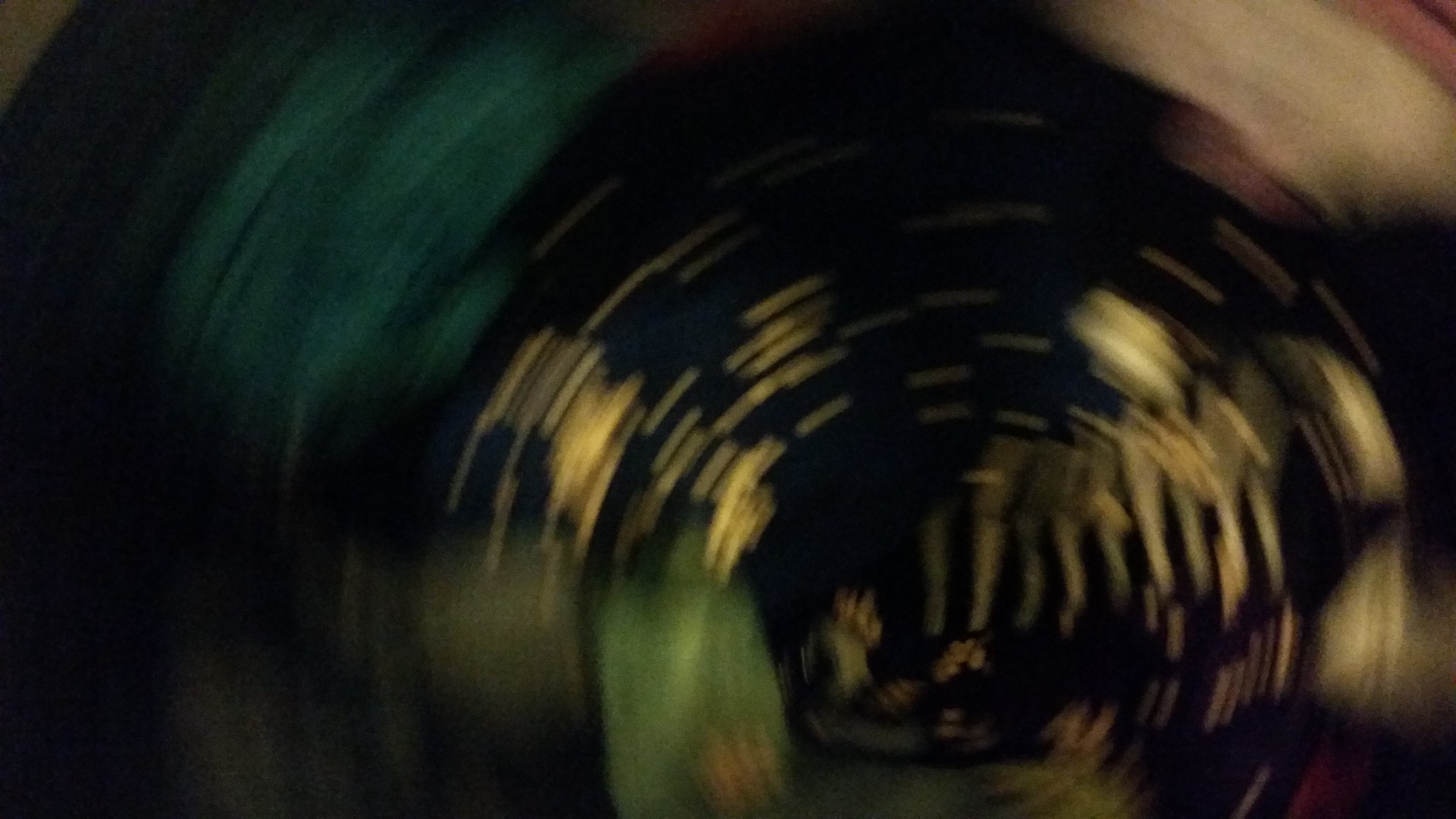This image, resembling a blurred painting, is an abstract display of swirling colors in a circular motion, evocative of water swirling down a drain with food coloring. The predominant color palette includes dark hues with bursts of vibrant tones. At the center, there's a mixture of yellow, light green, and dark blue hues, surrounded by an array of colors such as turquoise and off-white. The swirling pattern gets darker towards the outer edges, with prominent black and dark blue shades. As you move from the center outwards, the colors transition through greens, blues, and hints of reddish-orange on the right side. The entire image has a chaotic yet symmetrical feel, with circular motions creating a sense of spinning or movement. Details are blurred, making the image appear almost as if it were viewed through a fisheye lens or a photograph capturing rapid motion.